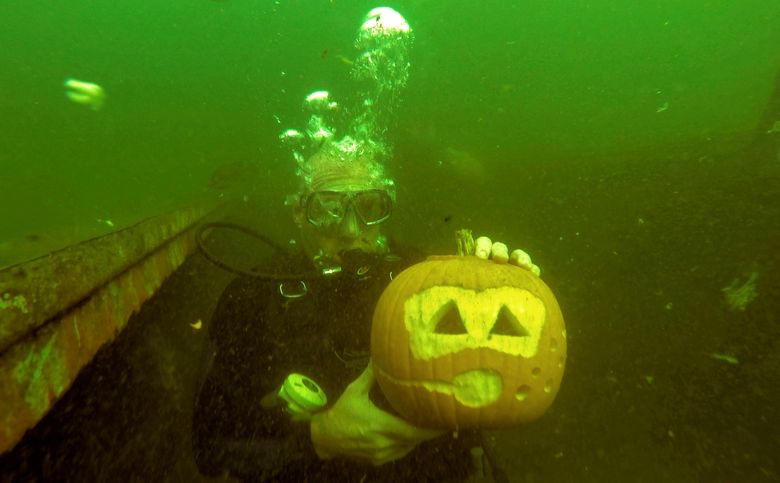In this underwater photograph, a diver is submerged in greenish-hued water, wearing a black dive suit, a mask, and a swim cap. The diver is grasping a jack-o'-lantern carved to mimic a diver's face, complete with a dive mask and respirator details, showcasing clever artistry. The water around him is filled with bubbles rising above his head, giving a sense of his recent motion. To his left, a long, rusty metal structure, possibly remnants of a shipwreck, adds a mysterious and adventurous element to the scene. The seafloor appears dark and barren, and faint outlines of small sea creatures, possibly jellyfish, are visible, enhancing the underwater atmosphere. The overall background transitions from a murky green at the top to a dirty brown at the bottom, creating a compelling contrast that frames the diver and his unique pumpkin companion.